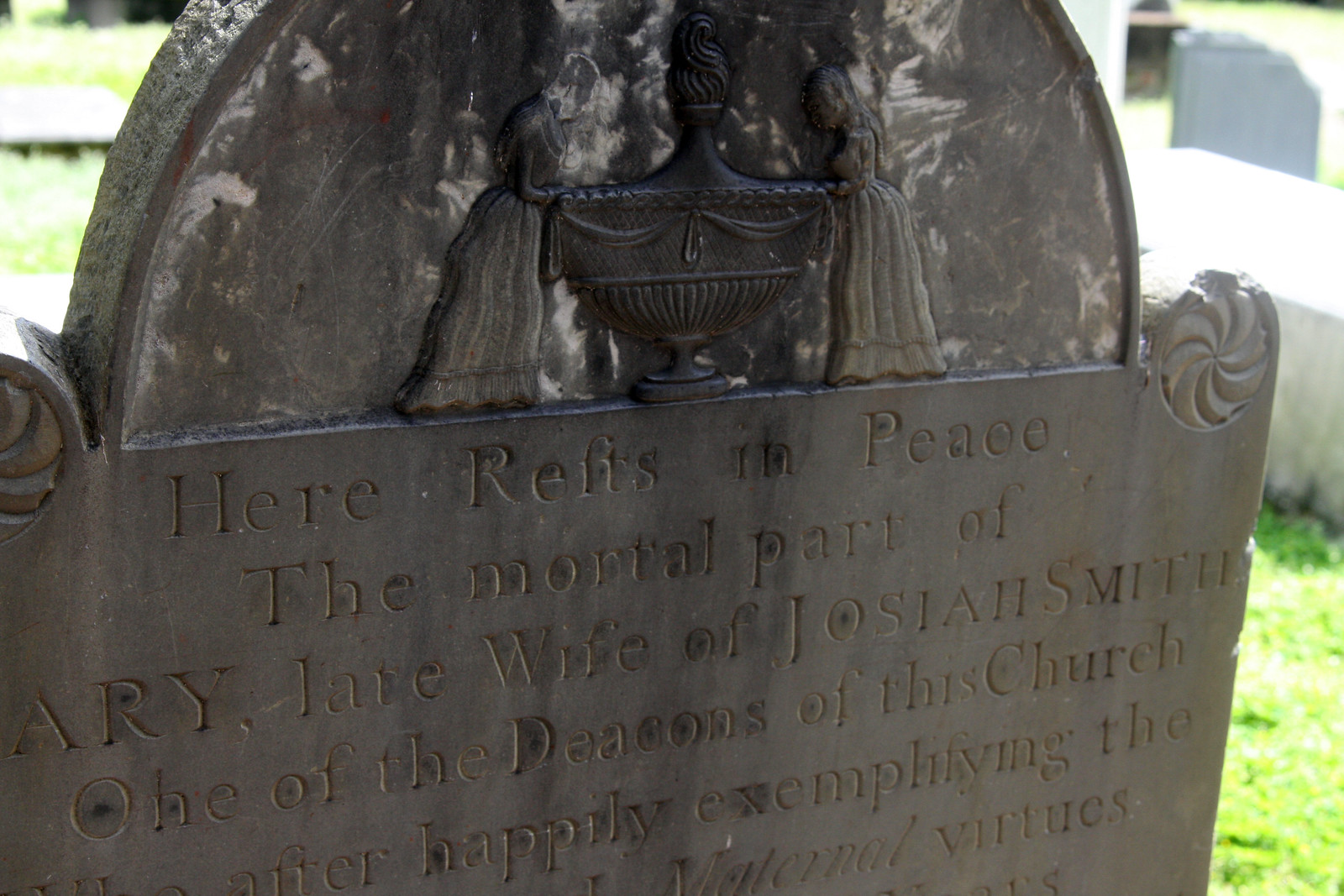This photograph, taken outdoors in the middle of the day, captures a close-up of an aged tombstone situated in a well-lit cemetery with grass and other headstones visible in the blurred background. The rectangular image prominently features the dark, scratched, and chipped arched gravestone in the center. The top of the gravestone is adorned with an engraving of two women standing over what appears to be a fountain or urn with flames. Below the engraving, the inscription, though partially worn and cut-off, reads: "Here rests in peace the mortal part of Airy, late wife of Josiah Smith, one of the deacons of the church. After happily exemplifying the maternal virtues..." The details reveal the tombstone's weathered state, with a mix of white, gray, black, and hints of orange colors forming a visually compelling snapshot of historic reverence.